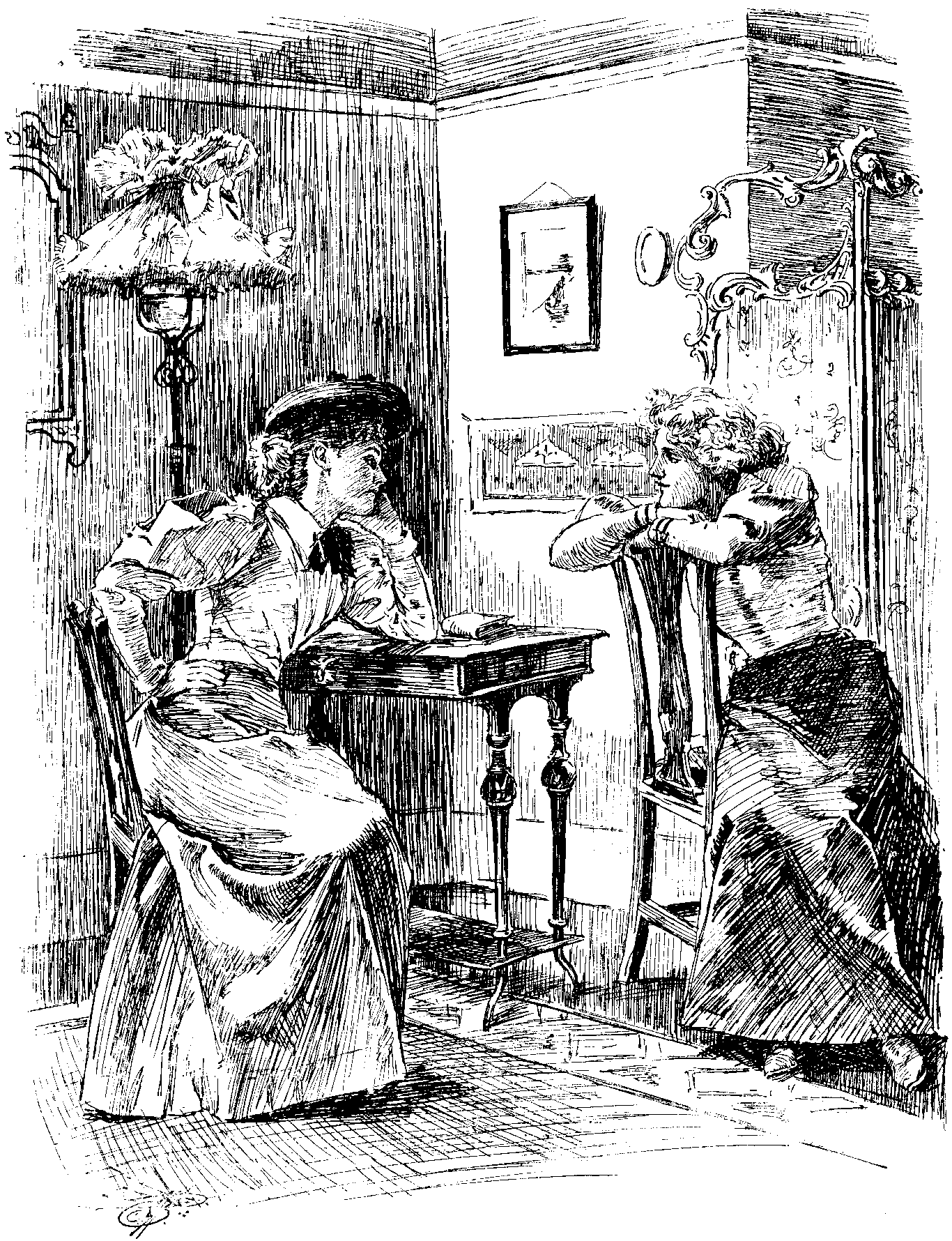The black-and-white hand-drawn sketch depicts an interior room setting from the 1800s, showcasing two women in period attire. The woman on the left, wearing a large black hat and a long dress with frilly sleeves, is depicted leaning on a small four-legged table with her elbow, as she rests her chin contemplatively on her hand. Opposite her, the second woman, also in a long dress but hatless, is seated sidestraddle on a chair, resting her chin on the backrest with her hands folded. The scene is richly detailed, with a lamp positioned to the left of the first woman, a framed picture on the wall, a screen curtain behind the second woman, and additional elements such as a mirror and a floor pattern enhancing the composition. The drawing, created entirely in pencil, captures the intimate and quiet nature of their interaction.